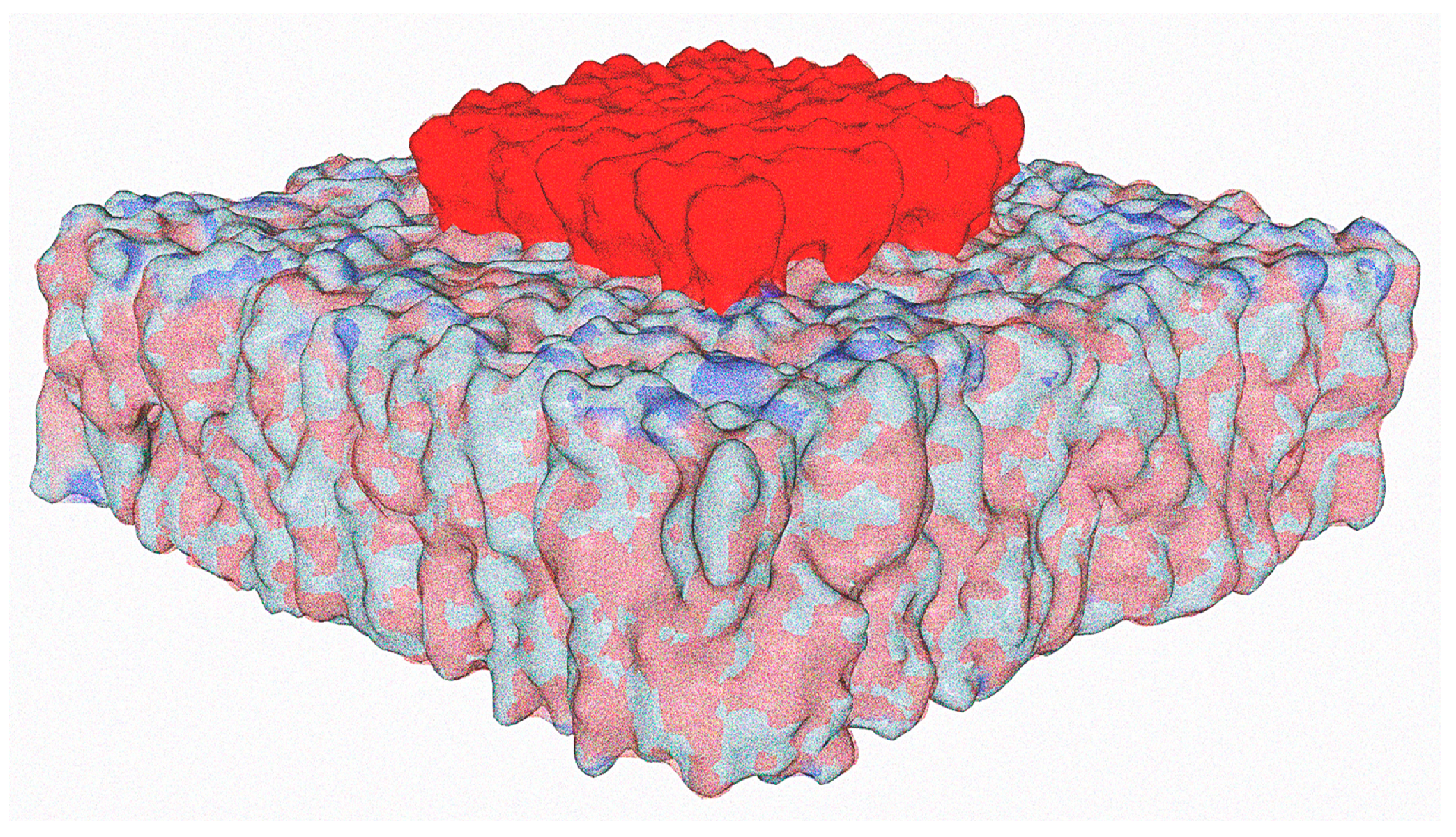The image is a detailed, abstract digital artwork featuring a three-dimensional model composed of two square-shaped layers set against a completely white background. The bottom layer is a larger diamond-shaped square with a complex camouflage pattern of muted colors, including dark blue, light blue, pink, and red, giving it a textured appearance similar to a spongy surface or mattress. Centered directly on top of this base layer is a smaller, solid dark red square that also has a spongy texture. The entire composition is oriented in such a way that the squares appear to be rotated, with their corners directed toward the viewer, making both the top and sides of each layer visible. This contrast between the vibrant layers and the stark white background adds to the striking visual effect of the artwork.